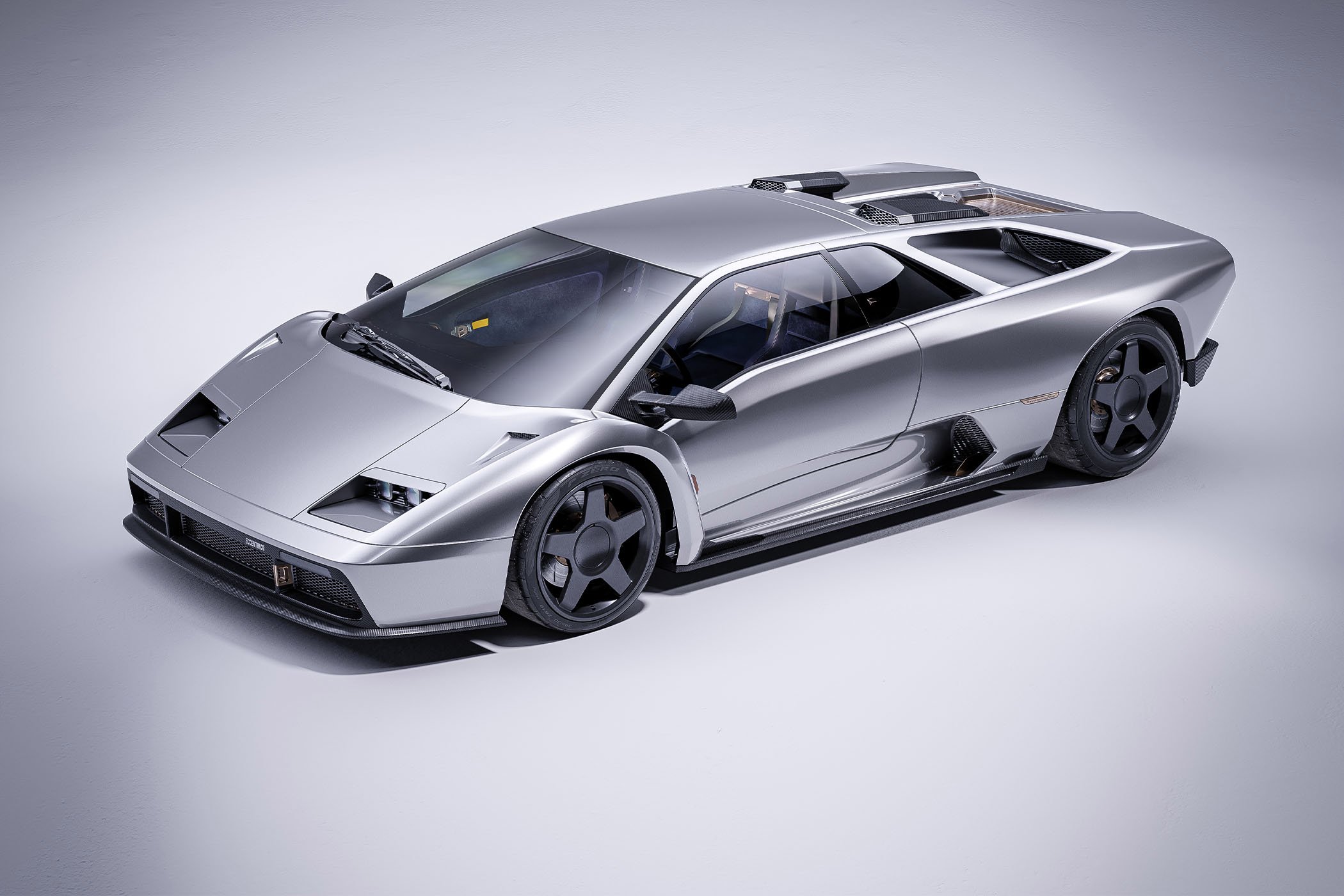This image features a detailed digital rendering of a silver Lamborghini Diablo with a sporty, souped-up appearance. The car, positioned front-facing towards the lower left corner and rear towards the upper right, is set against a minimalistic gray background that emphasizes its sleek design. The low-to-the-ground vehicle boasts black wheels and interior, with notable black racing scoops adding to its aggressive look. Red lettering adorns the side, though the specific text is unidentifiable. Notably, a small spot of yellow is visible inside the car, whose purpose remains unclear. Overall, the primary color palette of the image consists of various shades of gray and black, with touches of red and yellow adding subtle contrast. The realistic depiction, complete with racing gear, suggests it could be an exceptionally detailed toy model or a sophisticated digital concept.